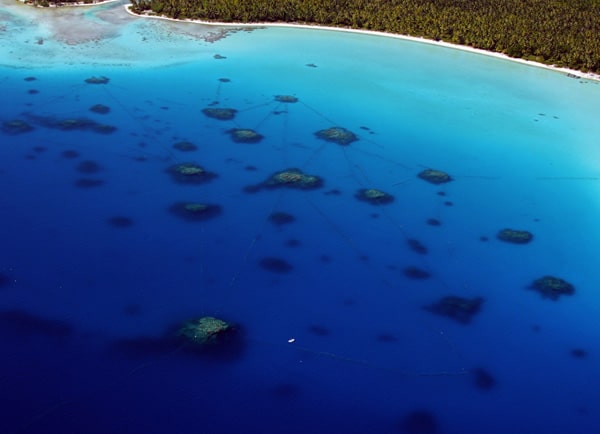The image captures a vast, mesmerizing body of water that appears to be a bay or an immense lake, characterized by its strikingly light blue, see-through clarity. The water, which dominates the majority of the photograph, transitions from teal near the right side to a deep cobalt blue towards the left. Within this crystalline expanse, patches of green seaweed and possibly submerged rocks can be seen, interspersed with other underwater growths creating a mosaic of green and golden hues beneath the surface.

Along the perimeter of the water, particularly at the top of the image, a thick, lush forest of trees frames the scene, with hints of white sandy areas around the edges. The forest is dense and wraps around the water, which itself flows and bends, suggesting the presence of additional land masses. These land masses include numerous green and golden patches of varying sizes, some large and prominent, others minuscule, dotting the lake and contributing to the complex beauty of the landscape.